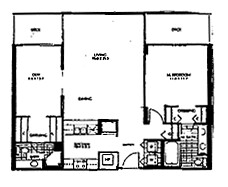This image depicts a floor plan of a rectangular house. Although the writing on the plan is small and somewhat illegible due to poor image quality, the layout is discernible. The house is organized into three rooms across and approximately three rooms down. 

Starting at the top, the top-right and top-left corners each contain two smaller rooms. Directly beneath these small rooms is another, slightly larger room. The focal point of the house is a large, central room that spans from the front to the back of the house. 

Moving down, there are additional rooms at the bottom of the plan, which include marked doors. One door, located at the bottom of the image, provides entry to the house and leads upwards before branching left, suggesting the presence of cabinetry or units. Similarly, there are more units to the right. In total, two doors in the plan indicate their direction of opening, while other rooms are accessible via open passages in the walls. Notably, the top-left and top-right rooms lack doors entirely.

The plan does not show any evidence of windows. The leftmost room features vertical lines whose purpose is unclear. The right room is densely packed with units, leaving no floor space or clear walking paths between them.